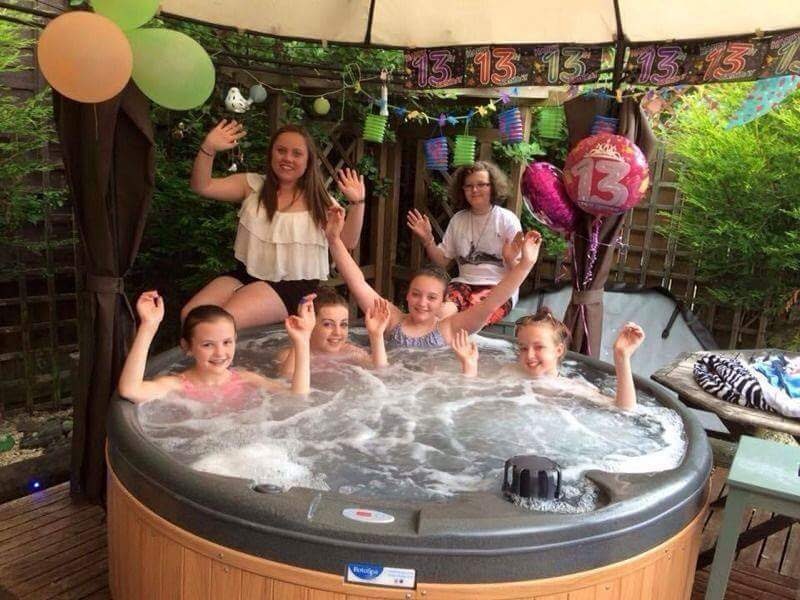This photograph captures a lively outdoor birthday party, likely celebrating a 13th birthday. Centered in the image are four pre-teen girls joyfully sitting in a gray and brown hot tub with the jets on, their arms raised in the air and bright smiles on their faces. They are joined in the background by two adult women, both dressed in white tops, one in a sleeveless white ruffled shirt with black shorts and the other in a short-sleeved white t-shirt with floral print pants. 

The covered porch area is adorned with festive decorations. The upper left-hand corner features three balloons—two green and one orange. A colorful banner stretches across the top, displaying the number "13" repeatedly in alternating colors of purple, orange, and green. Additional helium balloons, dark pink and light pink, with the number "13" inscribed in white, are positioned behind the girl on the far right.

The setting includes a light green square table in the lower right-hand corner and a larger wooden table to the right, which has towels or clothes draped over it, including a zebra-striped and blue towel. The entire scene is set against a backdrop of dense trees, providing a lush, green background that encapsulates the celebratory mood.